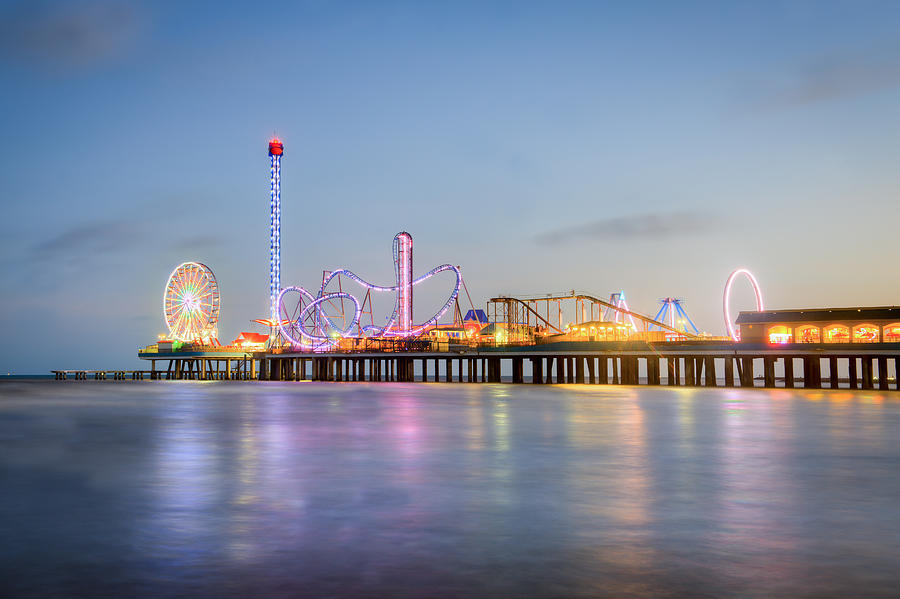This photograph captures a lively boardwalk carnival scene on a wooden pier extending into the tranquil ocean. The image, possibly taken during the early evening around 6 or 7 p.m., features a partly cloudy, grayish-blue sky that contributes to the serene backdrop. The pier stretches from the right side towards the left, stopping just before the left edge of the frame, and is filled with a vibrant array of amusement park rides. The ocean is remarkably still, perfectly reflecting the colorful lights of the attractions.

The focal point of the scene includes two prominent roller coasters: one with a noticeable pink or purple hue and another more traditional wooden coaster. A large ferris wheel, outlined in white lights, stands at the far end of the pier, while a towering drop ride with a red flame-like light at the top is prominently visible next to it. The amusement park also boasts swinging boat rides and several kiosks and stores lining the boardwalk. Additional rides and structures can be seen towards the back right of the image, adding depth to the bustling scene. The overall palette of the image is rich in blues from the ocean and sky, contrasted by the lively multicolored lights of the carnival rides, creating a dynamic and enchanting atmosphere.